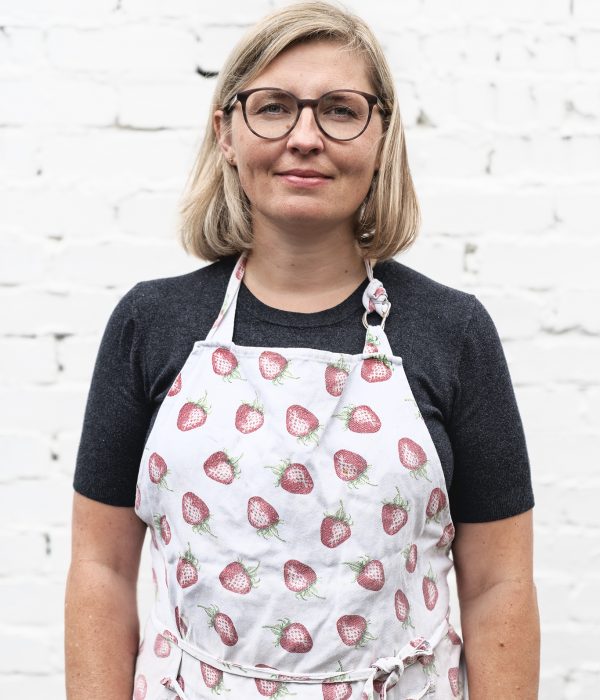In this photograph, the main focus is a fair-skinned woman with mid-length blonde hair, styled to her shoulders and side-parted on the right. She has glasses and wears a bit of makeup, along with a closed-lipped smile that exudes a sense of happiness. Her hair, gently tousled by the wind, complements her relaxed yet engaging demeanor. She is dressed in a gray to black t-shirt, over which she dons a white apron adorned with realistic-looking light red strawberries. Some strawberries have detailed seeds. The apron is tied in a bow on the lower right side of her abdomen. Behind her, the background features a blurry, painted white brick wall, accentuating the woman as the photograph's central subject. Adding to her distinct appearance, she has visible freckles on her fair arms and face, enhancing the natural and warm visual appeal of the image.